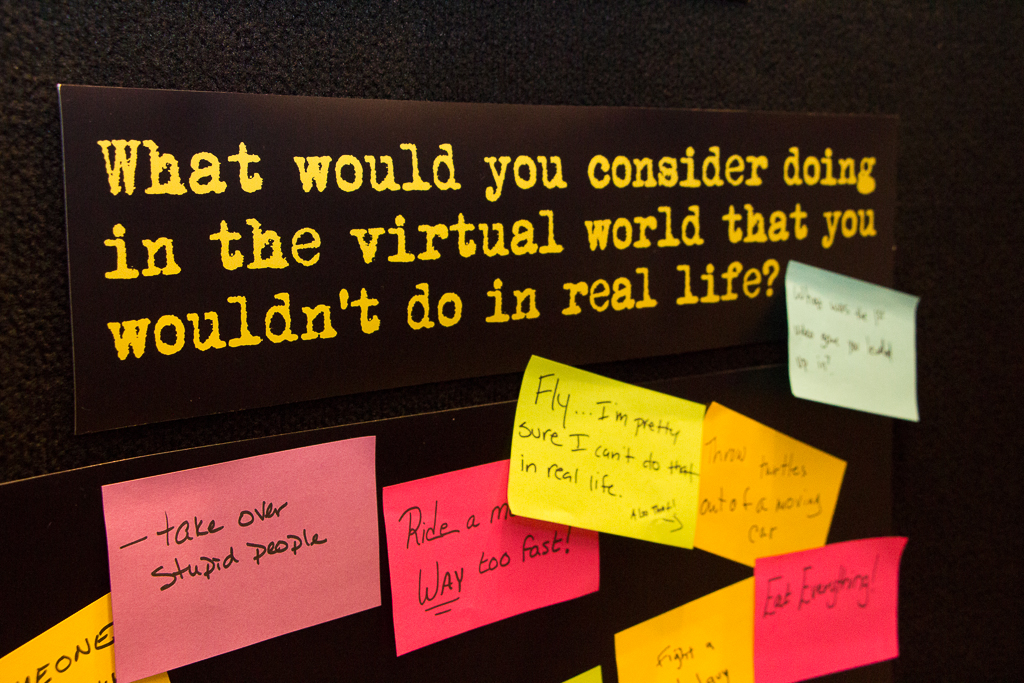The photograph showcases a black textured wall with a large, rectangular brown placard at the top. In bold yellow text, the placard poses a thought-provoking question spread over three lines: "What would you consider doing in the virtual world that you wouldn't do in real life?" Below this placard, numerous colorful sticky notes are posted, containing responses from various individuals. A prominent pink sticky note reads, "Take over stupid people," written in black magic marker ink. Another pink note says, "Ride a motorbike way too fast," with the word "way" underlined and capitalized. A yellow sticky note proclaims, "Fly, I'm pretty sure I can't do that in real life," and another pink note suggests, "Eat everything." There are additional sticky notes in various colors, including a blue one, but some are partially obscured or blurry, making them difficult to decipher.